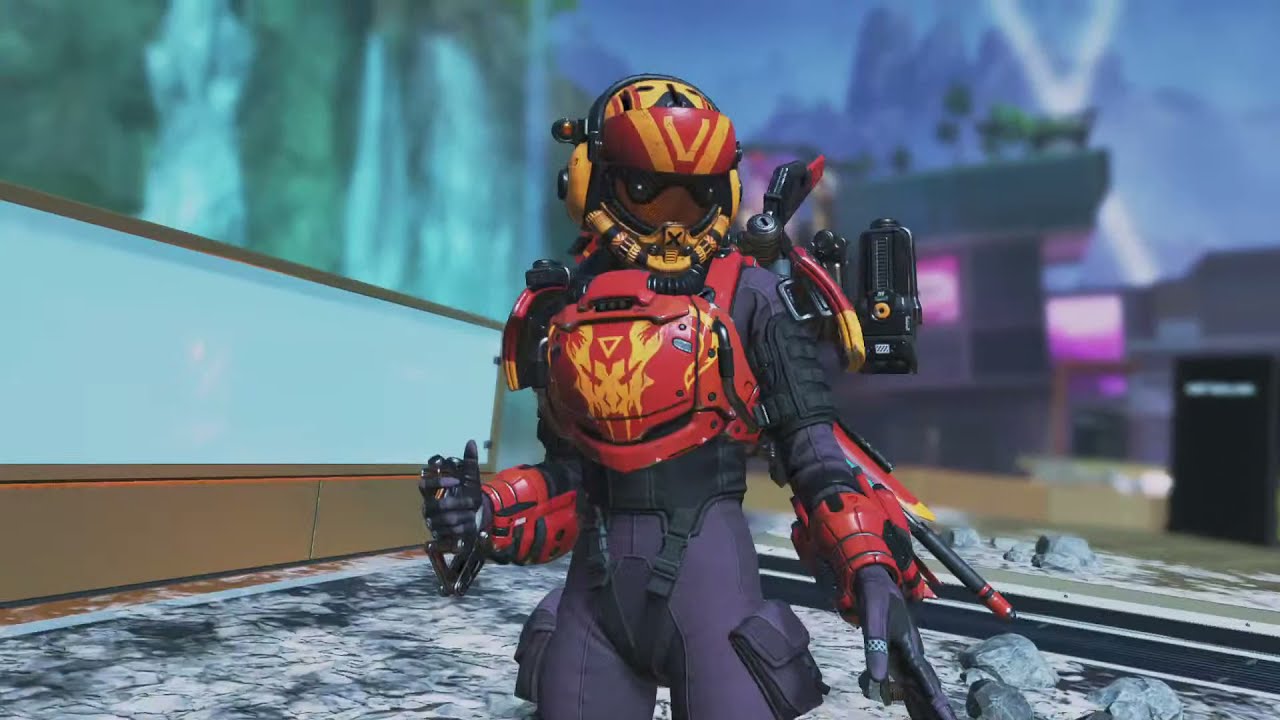In a vibrant, detailed digital rendering of a 3D video game, a central character resembling a transformer or anime fighter pilot commands attention. This armored figure, adorned in a striking mix of purple, red, yellow, and black, features a distinctive helmet reminiscent of an ant or bee with red and yellow stripes and a V-shaped design. The attire includes a red chest guard emblazoned with a demonic face and an upside-down triangle. One arm is outstretched, hinting at the gripping of a weapon, and the character appears ready for action with a potential jetpack attached.

The backdrop of this wide rectangular image is richly detailed. On the left side, a slightly diagonal wall transitions from light brown at the top and bottom to light blue and glossy in the center. Below, the multicolored, watercolor-like floor is interspersed with several gray rocks. In the upper left corner, blurred waterfalls can be seen, adding a sense of movement and life to the scene. The right side showcases a multi-story mansion, a striking contrast with its bright pink panels set against darker purple walls. This house emanates a violet light, intensifying the mysterious and fantastical atmosphere of the scene.